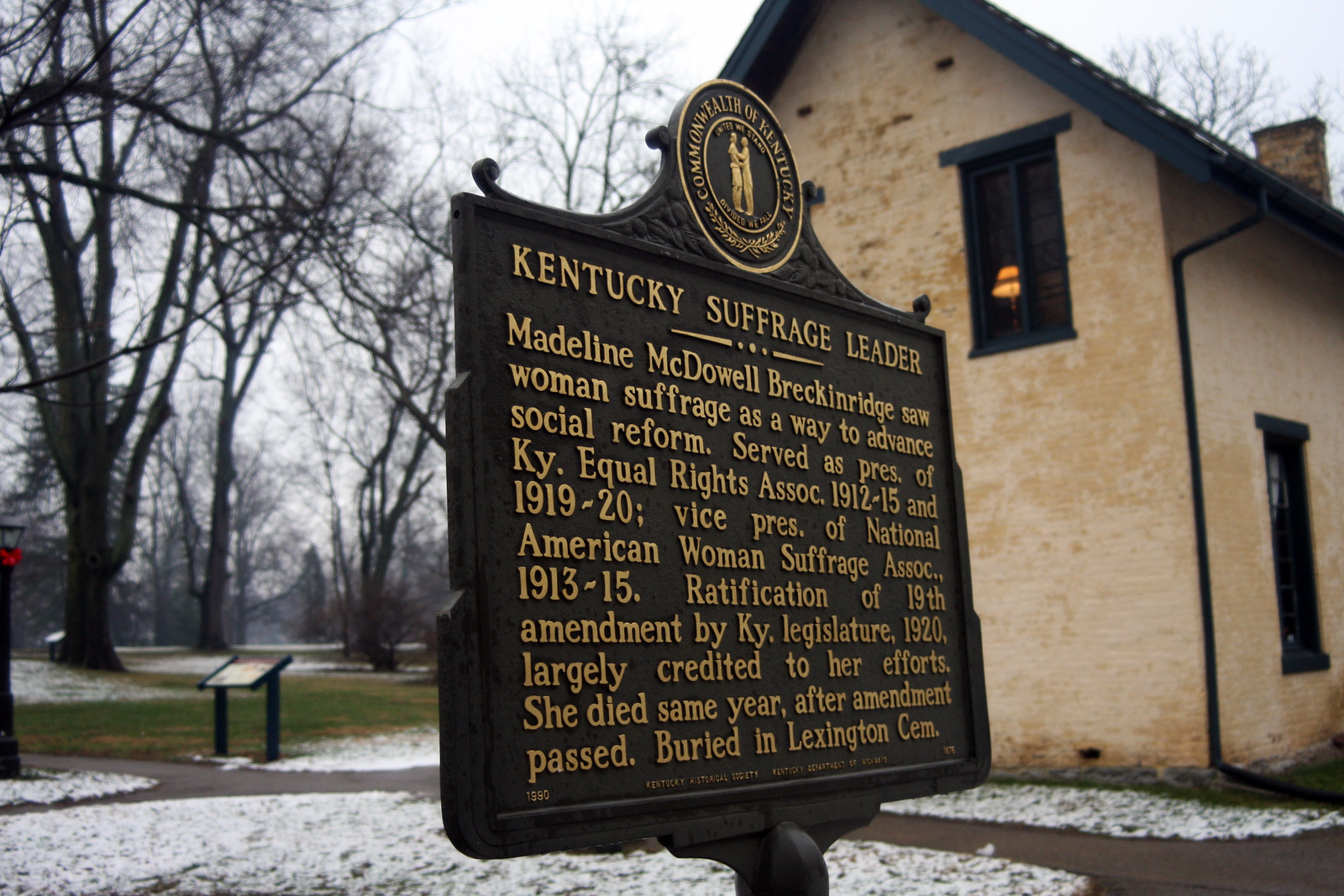The image depicts an historic house made of pale, aged bricks, appearing quite weathered and dirty. This two-story structure features windows framed in a dark blue trim, one of which has a lamp glowing warmly inside. The snowy surroundings include several cleared pathways winding through what seems to be a well-maintained and clean park. Tall, leafless trees stretch into the background with their lanky, bald branches. Centrally placed in the image is a black plaque with gold lettering under a gold circular logo that reads "Commonwealth of Kentucky," depicting two figures embracing. The plaque honors Kentucky suffrage leader Madeleine McDowell Breckenridge's contributions to social reform and women's suffrage. It details her roles: President of the Kentucky Equal Rights Association (1912-1915 and 1919-1920), Vice President of the National American Woman Suffrage Association (1913-1915), and credits her efforts toward the ratification of the 19th Amendment by the Kentucky Legislature in 1920. Sadly, she died the same year the amendment was passed and is buried in Lexington Cemetery. The house, likely now a monument, stands amidst a landscape of snow-covered ground and a few visible patches of grass, with the tranquil park stretching into the distance.